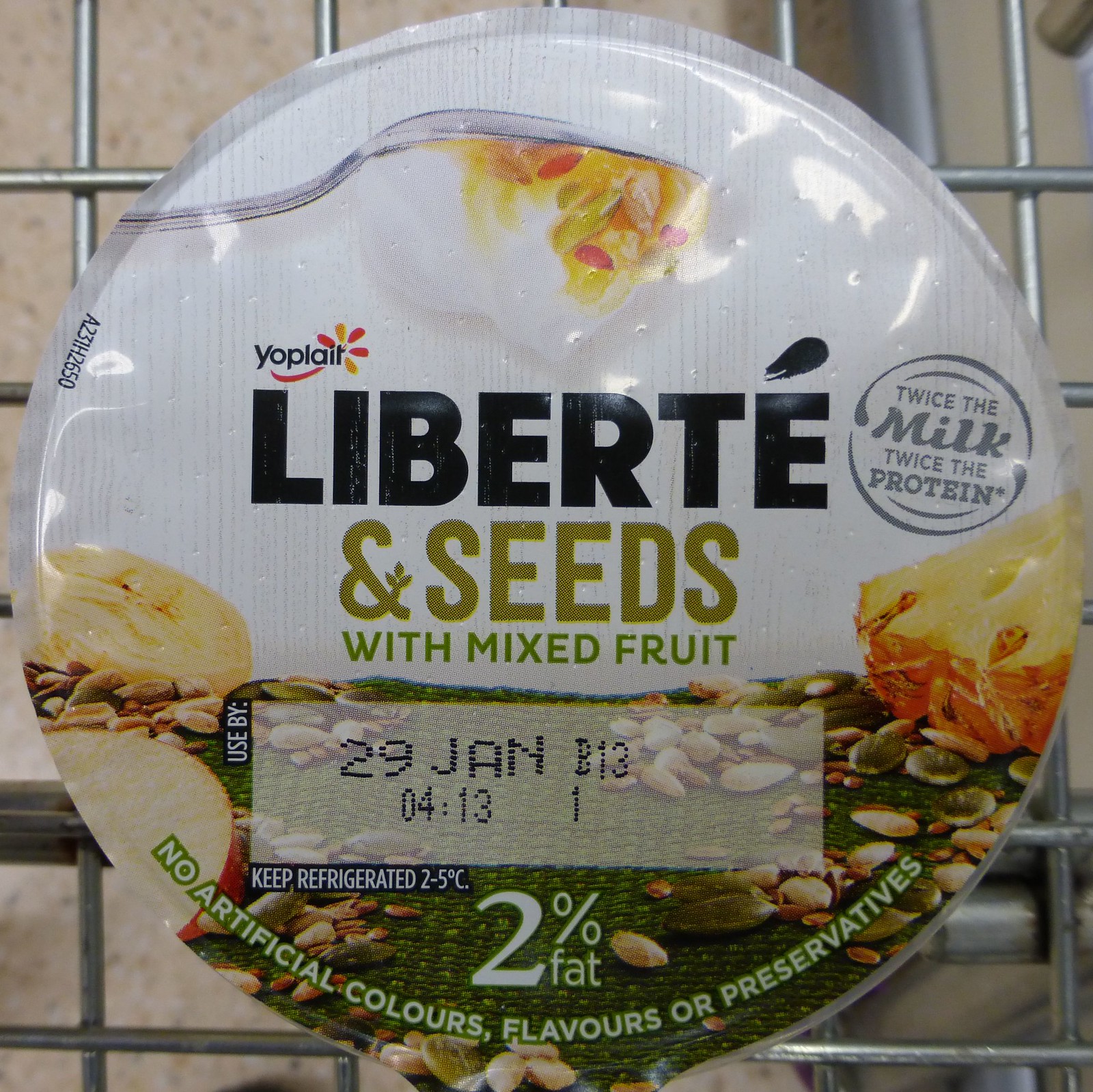This close-up photograph captures the top of a single-serve Yoplait Liberté yogurt container, resting on a metal wire grate. The lid is primarily white, featuring a spoonful of the yogurt held upside down at the top, which showcases the product's thickness as it does not fall off. In the center, bold black text reads "Yoplait Liberté," followed by "seeds with mixed fruit" in contrasting olive and green letters. A gray circle to the right bears the message "twice the milk, twice the protein." The lower half of the lid transitions into an image of various seeds and mixed fruits set against a green background. Detailed expiration information specifies "Use by 29 Jan, B13, 04:31," along with storage instructions indicating "keep refrigerated 2 to 5 degrees Celsius." Additional nutritional details state the yogurt contains "2% fat, no artificial colors, flavors, or preservatives." Beneath the container, the marble floor of a shopping cart, speckled in browns and tans, is partially visible through the metal wire of the cart.